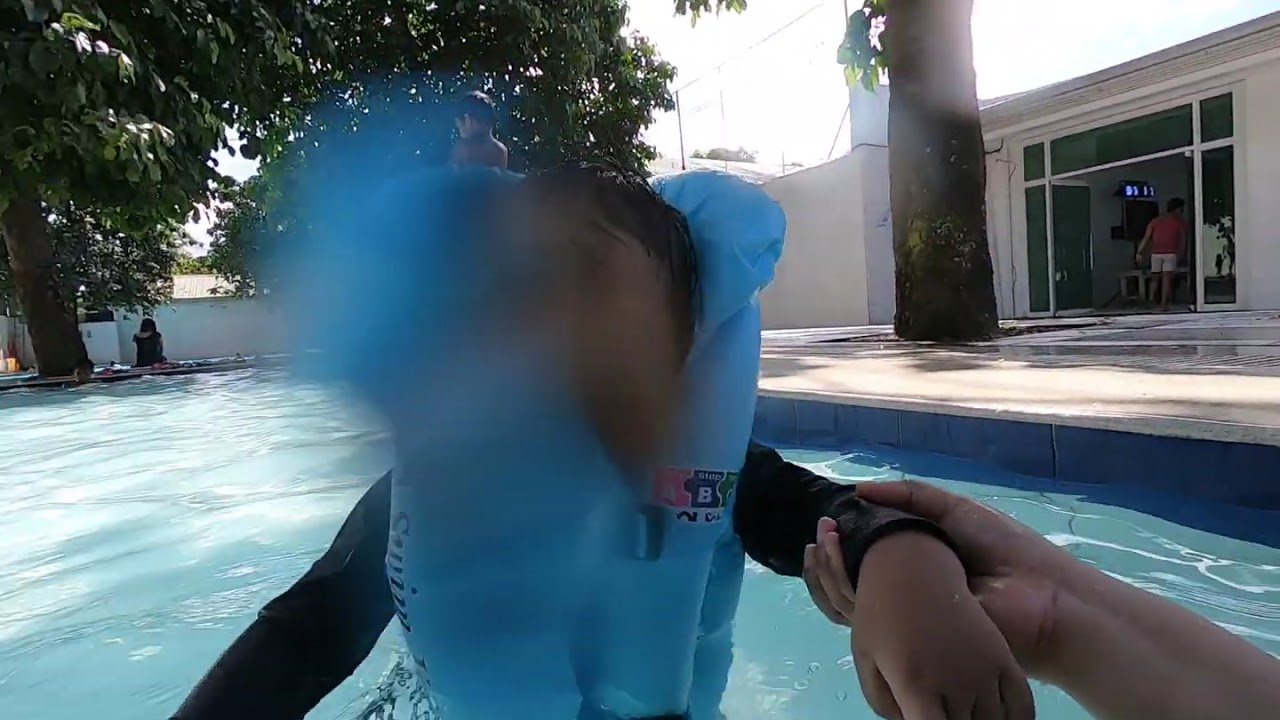In the center of the image, a young child wearing a blue life vest and a black long-sleeve swimming suit is positioned in a swimming pool, being held by the hand of an adult whose arm extends from the bottom right corner of the photo. The child's face is notably replaced with that of a bird, adding an unusual twist to the scene. The pool itself is light blue, bordered by darker edges, and is surrounded by beige pavement. To the right side of the pool, a house with white walls and a flat roof features a large windowed entrance, where a man in white shorts and a white and red top is visible, appearing ready to step outside. Behind the pool, a large tree trunk rises, its branches providing a canopy over the scene. Additionally, another child stands in the background on the pool deck.